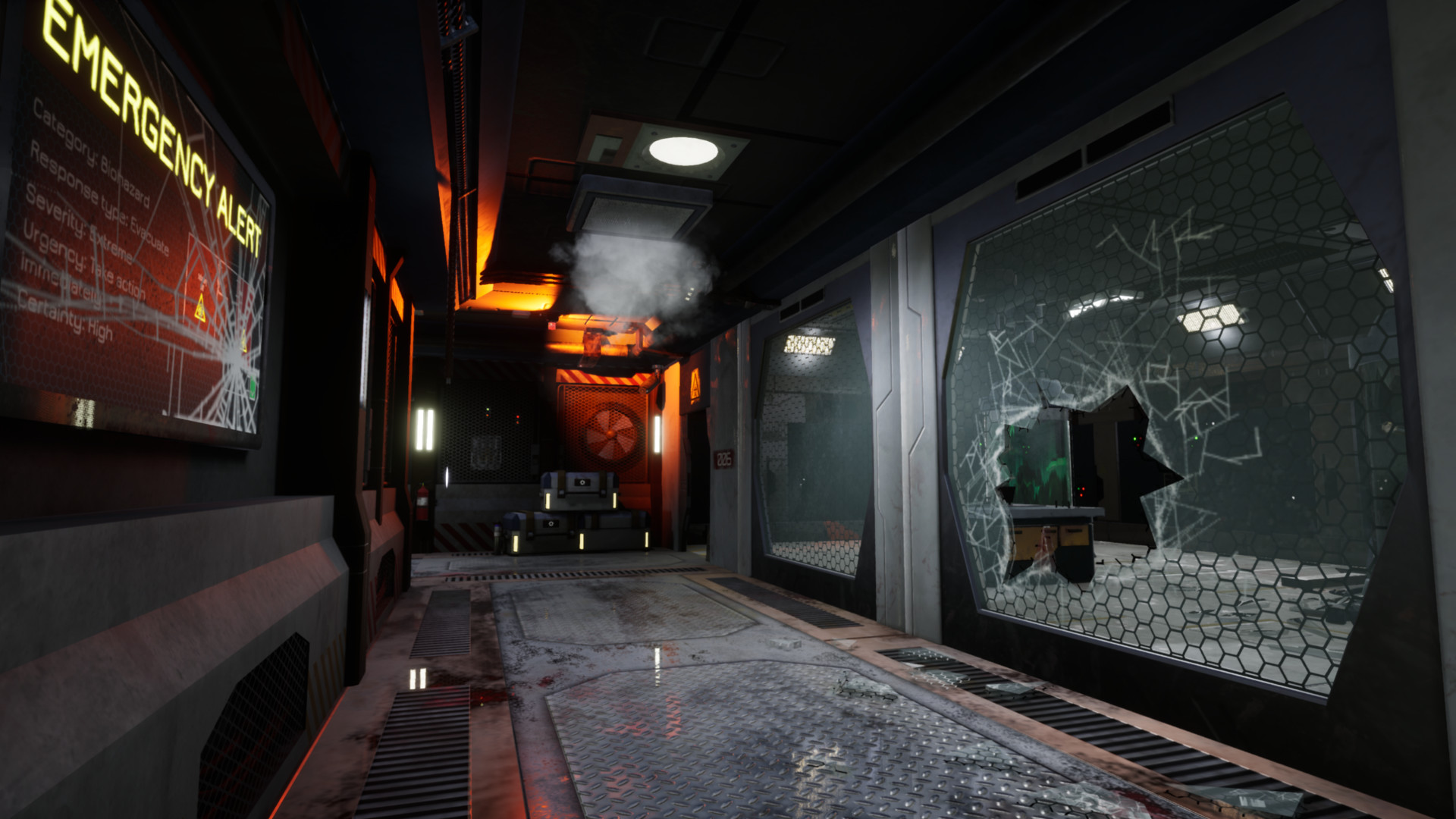The image captures a dark, ominous hallway that appears to be from a video game or movie set, possibly an abandoned or dangerous facility. The scene is primarily lit by a round overhead light, casting just enough illumination to reveal key details. The floor is made of metal grating, with vents lining the sides. On the left-hand side, there's a large, cracked screen displaying the words "Emergency Alert" in yellow; the screen bears a broken, spiderweb-patterned crack. Opposite the screen, the hallway features full wall-to-ceiling windows reinforced with steel; one of these windows is shattered, leaving a jagged hole through which a dark, indistinct room can be seen, possibly containing a tank or machinery on a desk. Towards the end of the hallway, smoke is seeping from an open vent on the ceiling. The entire scene is permeated with an eerie atmosphere, heightened by the presence of other lights and a danger signal in the distance. The setting is primarily composed of dark gray, steel, and black tones, contributing to the unsettling, foreboding environment.